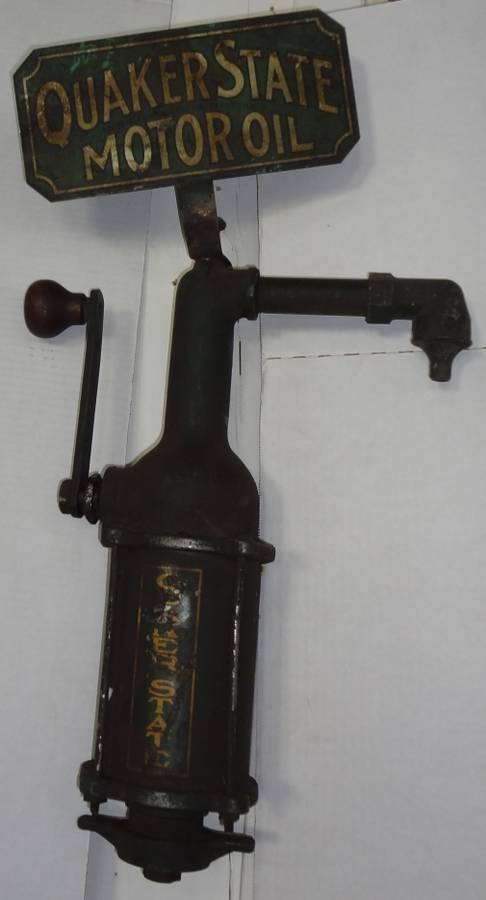The photograph depicts an antiquated, metallic instrument primarily black in color, likely constructed from metal or steel. This device features a cylindrical body with a pipe emerging from the top, bending outward. On the left side of the cylinder, a handle or crank is visible, and the instrument terminates in a bell-like bottom. Affixed to the top is a dirty, forest green metallic board inscribed with “Quaker State Motor Oil” in faded yellow and brown text. The cylindrical surface also bears the words "Quaker State" in yellow, although these are not very clear. The background consists of a white wall, adorned with vertical wooden planks and a slight crack on the right side. The sign is slightly tilted to the left, contributing to the vintage and worn-out appearance of the entire setup.